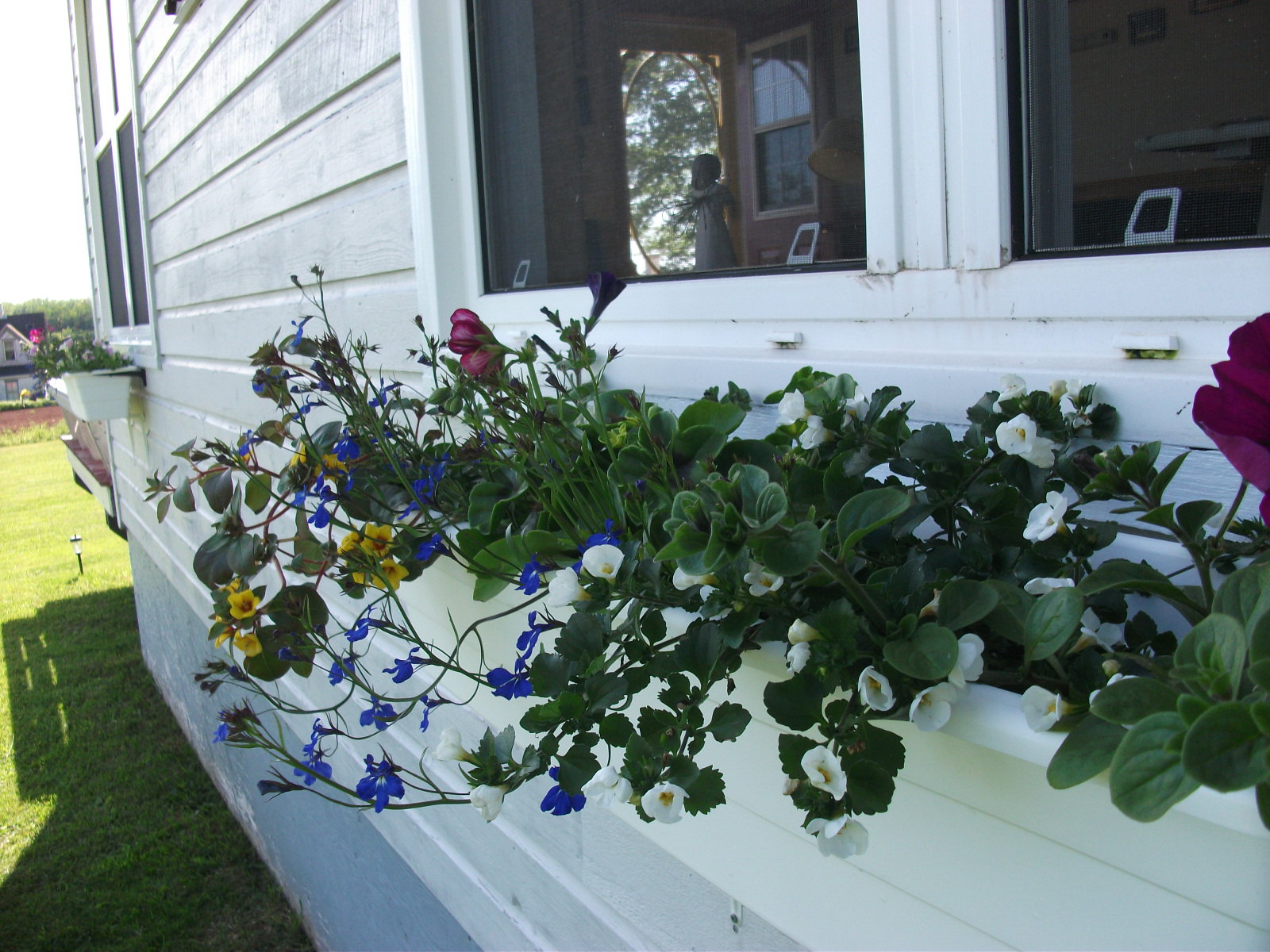This photograph captures the side of a somewhat old-fashioned, white-wood-paneled house, situated in a well-tended suburban neighborhood. The photo appears to have been taken on an overcast midday, casting a gentle, diffused light over the scene. Below the two side windows, there are garden shelves, or mantels, hosting a vibrant array of flowers, including red roses, white, yellow, blue, pink, and purple blossoms, all thriving in their pots and adding a colorful touch to the white siding.

Glancing through the windows, one can make out minimal interior details, such as a door opening, a table, a lamp, and some wall-mounted pictures and paintings, although visibility is somewhat obstructed by a net covering on the windows, casting a shadowed effect. In one of the windows, there's a faint outline of what appears to be a doll or similar object, positioned as if floating near the door due to its height and placement.

The grass in the foreground is lush and green, adorned with lawn lights, signaling meticulous lawn care. Across the street on the left, the presence of other houses underscores the suburban setting, creating a scene of serene, everyday beauty.